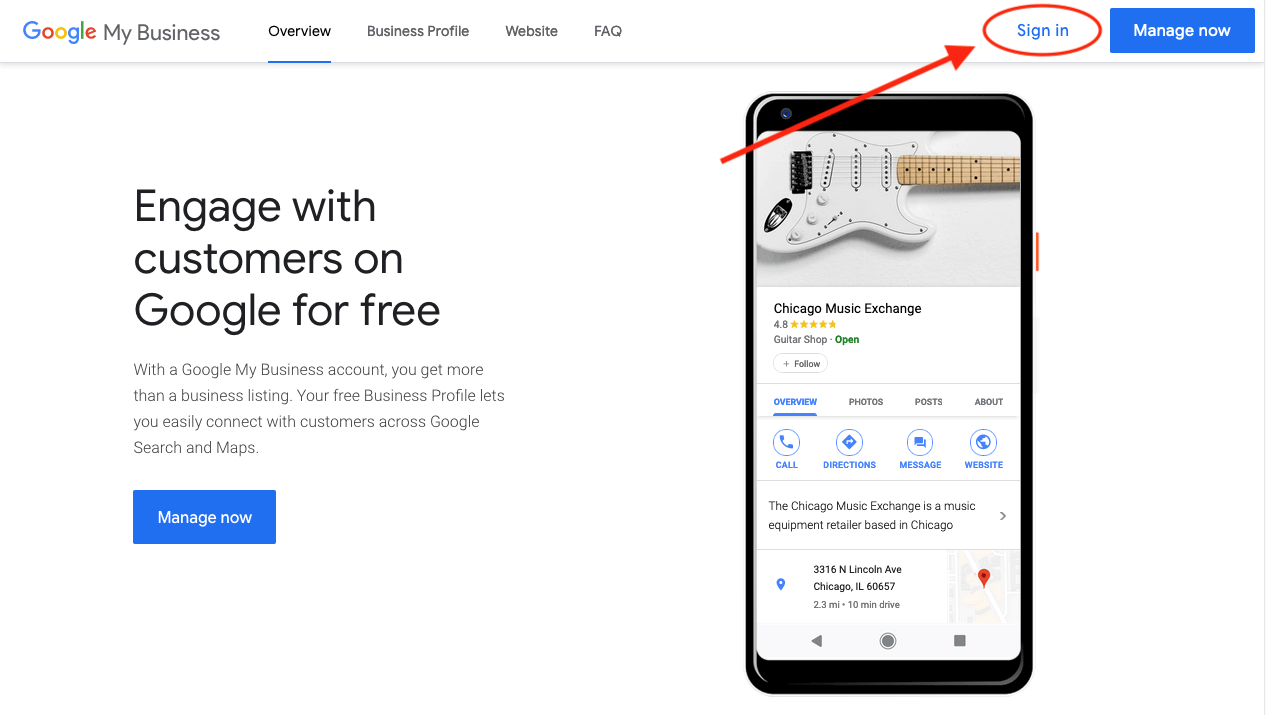The image displays a screenshot of a "Google My Business" interface against a white background. 

At the top left, there is a navigation menu with the "Overview" tab highlighted in blue. The adjacent tabs are "Business Profile," "Website," and "FAQ." 

On the top right, the word "Sign In" is encircled in red with a red arrow pointing towards it, drawing attention to the login option. Below this, there is a blue button labeled "Manage Now."

The main content of the page features a large headline in bold, stating "Engage with Customers on Google for Free." Below, there's a descriptive paragraph: "With a Google My Business account, you get more than a business listing. Your free business profile lets you easily connect with customers across Google Search and Maps."

Under this text, another "Manage Now" button is prominently displayed.

Centered on the screen is the profile of "Chicago Music Exchange." An image of a white guitar with a light wood-colored neck is shown. The profile has a rating of 4.8 stars. 

Tabs such as "Overview," "Photos," "Post," and "About" are listed beneath the profile picture, with "Overview" underlined in blue, signaling it as the current view. 

Below the tabs, there are four action buttons in blue: "Call," "Directions," "Message," and "Website."

Further down the profile, detailed information about "Chicago Music Exchange" is provided. It is described as a music equipment retailer located at 3316 Lincoln Avenue in Chicago, 2.3 miles away.

The image overall captures the layout and functionalities of the Google My Business profile, with a specific spotlight on the "Chicago Music Exchange."